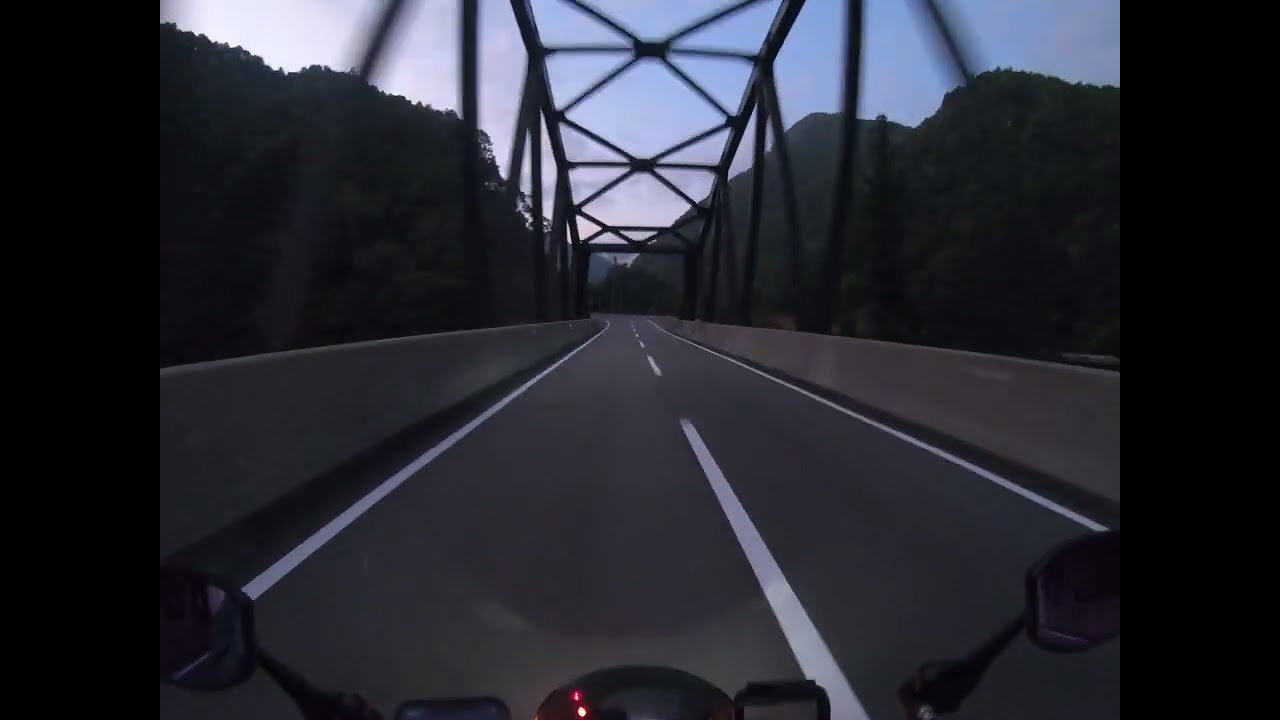This color photograph, taken from a GoPro mounted on the helmet of a motorcycle rider, captures an immersive point-of-view shot as they travel on a bridge section of a two-lane highway. Both the rearview mirrors and the front edge of the motorcycle are visible in the bottom corners, emphasizing the dynamic experience. The motorcycle is positioned in the left lane on the dark gray, paved road, which features a white broken center stripe and white striping on either side. Concrete walls line the edges of the road, accompanied by a trestle-like metal structure overhead. In the distance, the road disappears into a horizon framed by blue sky and dense forests on either side. The photo's motion and framing suggest the swift movement of the rider, further enhanced by the blurry depiction of the overhang above. The overall scene is a realistic, detailed snapshot from a GoPro video, capturing the essence of a motorcycle journey through a scenic yet structured environment.